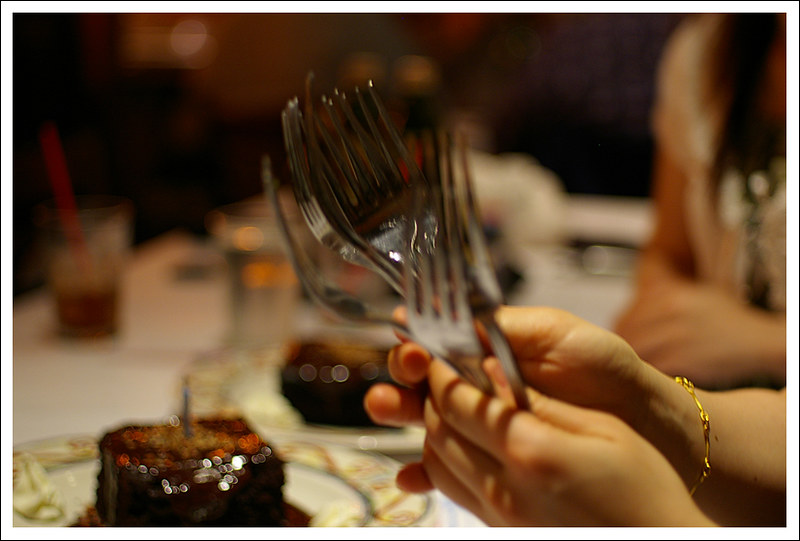This indoor color photograph captures the profile of an individual handling a collection of approximately 12 to 13 clean, silver dinner forks. The focus is on the person's hands, which enter the image from the lower right. The right wrist features a beautiful gold bracelet. The forks, held in both hands with the tongs pointing up, suggest a meticulous gathering or laying out process. The blurry background depicts a table setting: a plate with a chocolate cake adorned with a single candle, partially visible on the left, accompanied by a glass with a red straw. In the upper right background, another person's blurry hand is slightly distinguishable. The entire scene is set against a dark upper backdrop, emphasizing the silver forks and the gold bracelet as focal points.